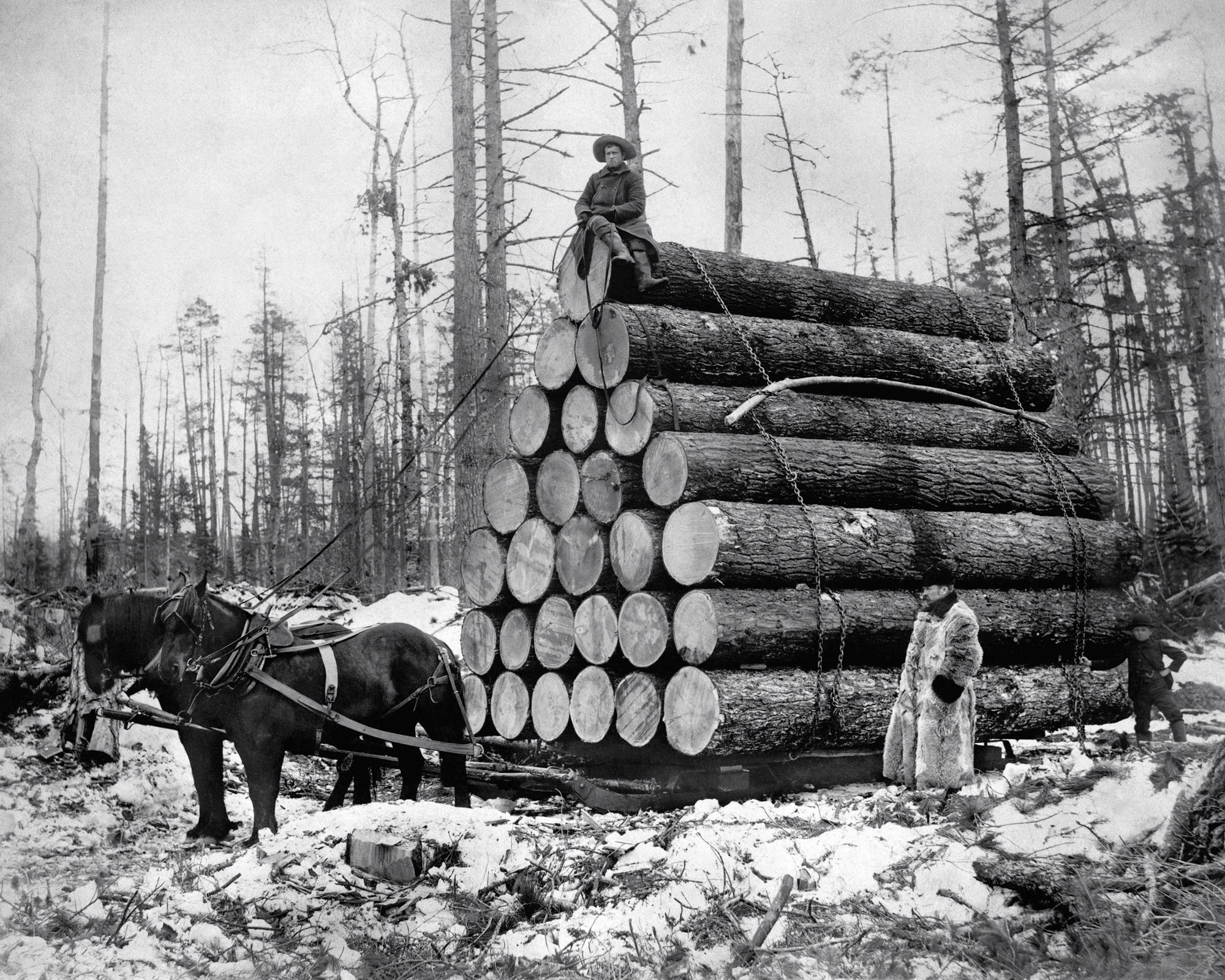A black and white photograph captures a poignant scene of a logging team working through a wintry forest. The central focus is a large, pyramid-shaped stack of logs, carefully arranged with six logs on the bottom, another six on the next tier, followed by five, then four, three, two, and a single log on top. The logs are tightly secured with metal chains, and the entire stack rests on a flat sled.

At the pinnacle of the log pile, a man sits, dressed in a long jacket, boots, and a hat, holding the reins connected to two dark-colored workhorses standing at the front of the sled. The ground around them is lightly dusted with snow, adding to the somber, overcast atmosphere depicted in the image.

To the right of the log stack, a man in a heavy, fur-lined coat and a black hat stands, appearing to inspect the arrangement. In the background, a young boy dressed in a long, dark suit with a hat and boots is seen, holding onto one of the chains. The surrounding trees are bare, their leafless branches silhouetted against the hazy, cloudy sky, highlighting the harshness of the winter setting and the rugged nature of their labor.